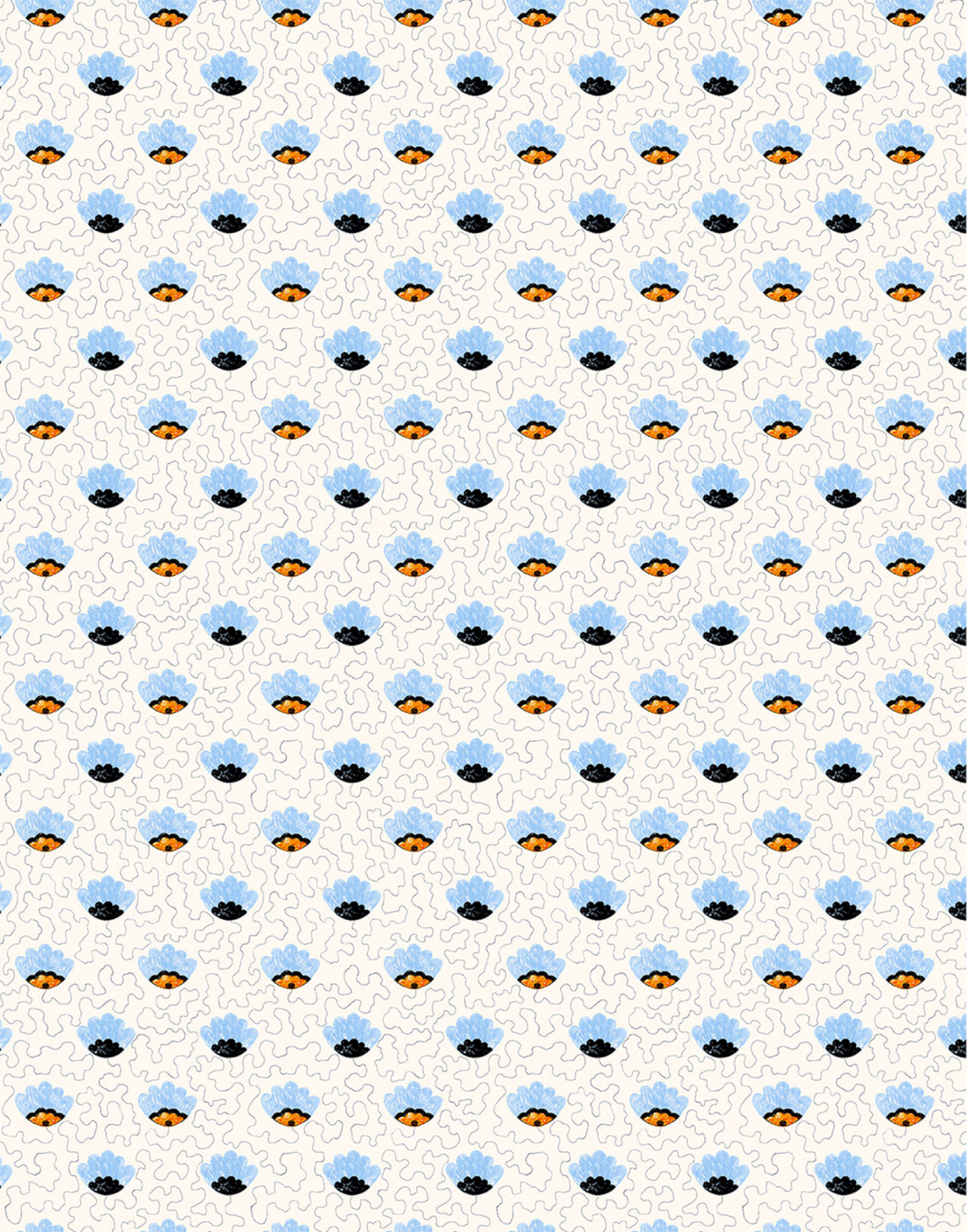The image features a seamless pattern resembling potential wallpaper, characterized by a cream-colored background with subtle blue lines creating a lattice-like grid. Overlaying this background is a repetitive design that alternates between gold-colored and black-colored dimple shapes, each resembling a small crown or bead with distinct detailing. The golden dimples have intricate black outlines and dots at the center, while the black dimples are simpler, with no additional coloring. This pattern alternates diagonally, creating a dynamic and visually engaging design that could serve purely decorative purposes, making it suitable for applications such as wallpaper, wrapping paper, or other decorative surfaces.